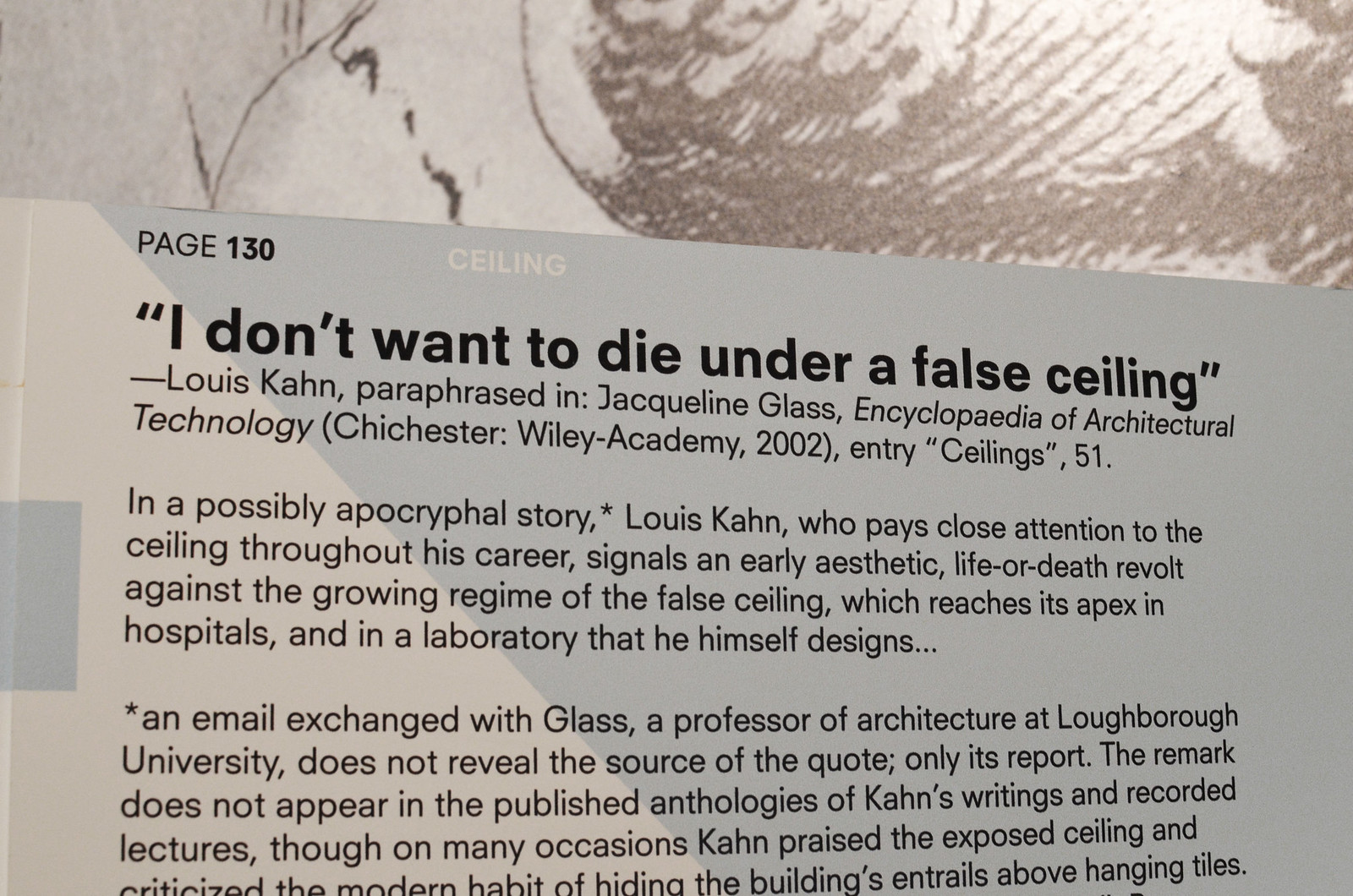A white sign in the foreground, framed by a light gray background and a silverish shape, perhaps a ball, displays an excerpt from "Jacqueline Glass Encyclopedia of Architectural Technology." The top of the sign reads "Page 130," followed by a bold quote, "I don't want to die under a false ceiling," attributed to Louis Kahn. The sign elaborates that this quote, possibly apocryphal, reflects Kahn's early revolt against the widespread use of false ceilings, particularly noting their prevalence in hospitals and laboratories, including one he designed. The text mentions that Louis Kahn's close attention to ceilings throughout his career signaled his aesthetic stance against the modern trend of concealing building infrastructure with false ceilings. This detailed passage is framed within the context of entries from Chinchester Wiley Academy, 2002, entry "Ceilings 51."